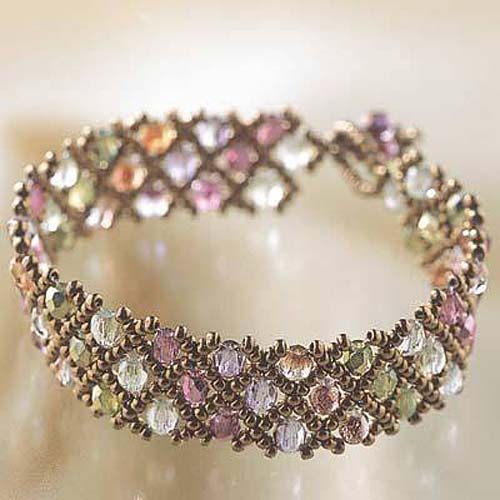The image features a sophisticated bracelet with a distinctly thick band that radiates elegance. This bracelet is adorned with an array of sparkling gems in pastel hues, including light purple, light orange, light green, white, and a subtle pink. The gems are intricately set within a crisscross pattern of metal, reminiscent of diamond shapes, adding to the intricate design.

The bracelet is showcased on a reflective, gold-toned, shimmering surface that beautifully enhances the sparkle of the gems. The clasp is visible at the back, suggesting that the bracelet is open-ended and does not form a complete circle. The band of the bracelet itself glistens under the light, complementing the radiant gems and adding a final touch of luxury to the piece. This bracelet exudes a sense of stylish refinement and is designed to be a standout accessory.